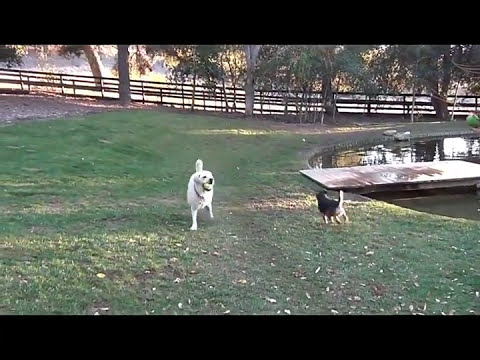The image depicts two dogs energetically playing outdoors in what appears to be a private property, possibly a farm. The scene is set in a well-maintained, but slightly drying grassy area next to a small, round pond, complete with a wooden dock extending into the water. The surrounding landscape features a long wooden fence lined with trees that provide ample shade, suggesting it's midday but without harsh sunlight. The white dog, which looks like a Golden Retriever, is at the center of the action, holding a tennis ball in its mouth. It seems to be barking or in the midst of playful activity. In contrast, a smaller dog with brown and black coloring is seen running towards the white dog, likely eager to join the play. The image quality gives a nostalgic feel, reminiscent of a screen capture from a VHS tape, with black horizontal bars visible at the top and bottom. Despite the low resolution, the dynamic interaction and joyful movement of the dogs are clearly conveyed.